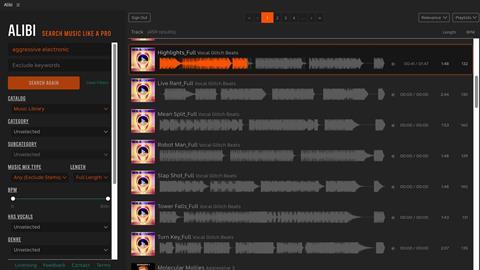This image, sourced from the Alibi website, features a sleek, all-black background. Dominating the upper left corner is the Alibi logo in white, accompanied by the slogan "Search music like a pro" in vibrant orange. Below the slogan, an orange search button is prominently displayed, along with various filtering options such as Catalog, BPM, Genre, and Max Vocals, facilitating an efficient search experience.

Moving towards the upper center section, a page navigation bar is visible, offering a straightforward mechanism to cycle through and skip between different pages. Beneath this, the interface showcases sound waves and audio clips, with the topmost clip currently being played, indicated by the orange highlight over the gray sound wave bars. The subsequent sound wave bars remain in a muted gray, awaiting selection.